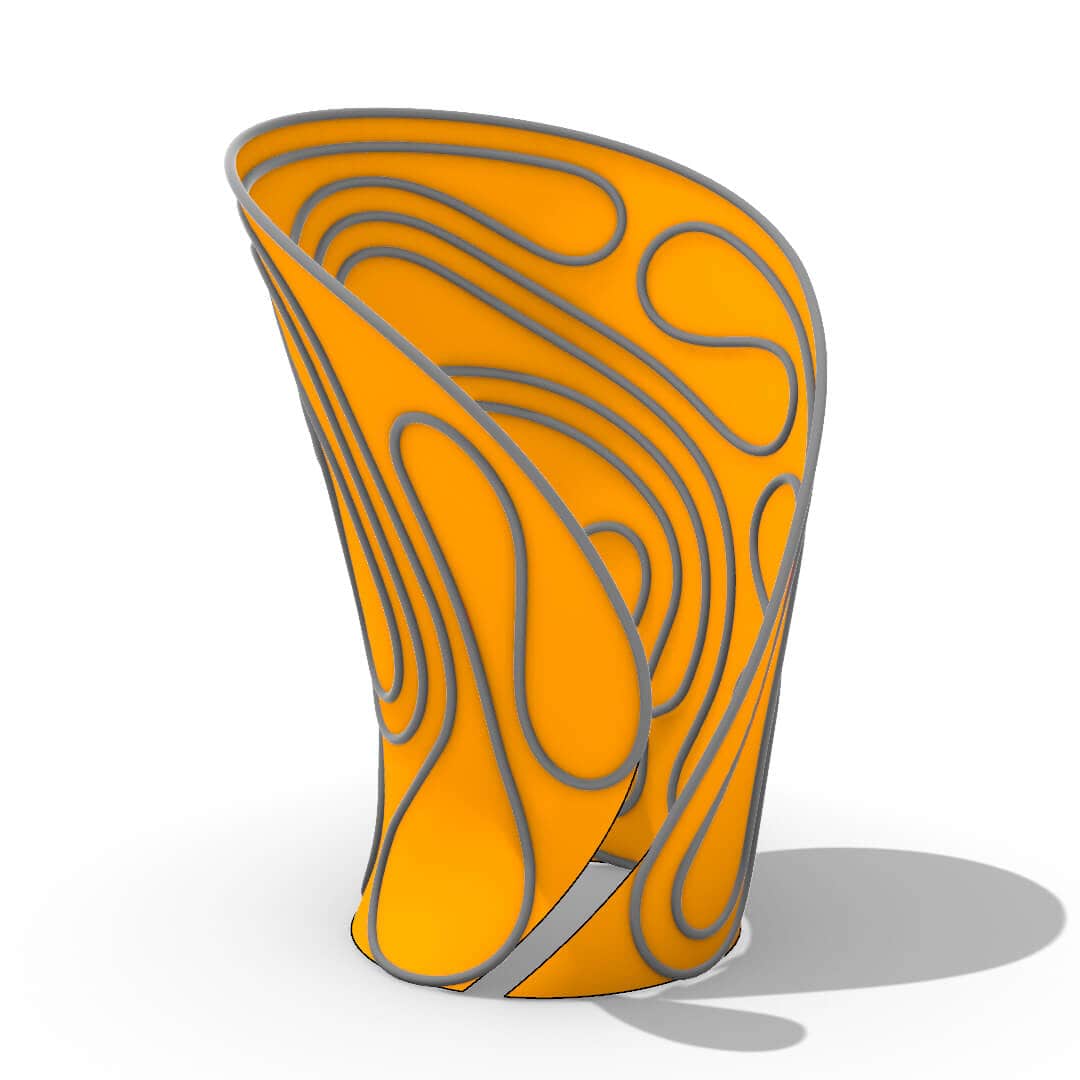The image features a bright orange object, potentially resembling a lampshade, bracelet, or unconventional piece of headgear. The object, possibly made of silicone, stands upright on a plain white and grey platform and measures several inches in height. It exhibits a wider top that gradually narrows towards its circular base. The sides and top of the item are curved, with slits incorporated into its design. Encircling the orange surface are several grey lines or silver wiring that swirl and wrap around the object. A noticeable shadow extends to the right and also appears inside the partially open structure, adding to its three-dimensional appearance.